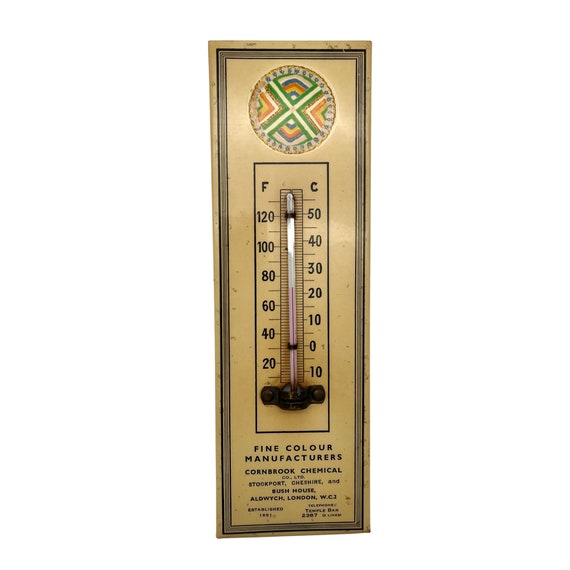This photo features a vintage wall-mounted thermometer, likely from a promotional piece distributed by a business. The thermometer is encased in a brass rectangular frame, with a cream-colored enamel backing. The central feature is a glass mercury thermometer with a black rectangular border and a thin glass tube, where the red mercury indicates a temperature around 70-72 degrees Fahrenheit (approximately 23 degrees Celsius). The temperature scale shows Fahrenheit on the left, ranging from about 15 to 125 degrees, and Celsius on the right, ranging from about 10 to 55 degrees. Above the thermometer, there is a multicolored, circular crest with a cross motif, reminiscent of an Indian-style logo. Below the thermometer, there is faded writing that reads, "Fine Color Manufacturers, Cornbrook Chemical, Cheshire," using the British spelling of "color." This craftsmanship and design suggest that it is a collectible advertising piece, designed to be both functional and decorative.